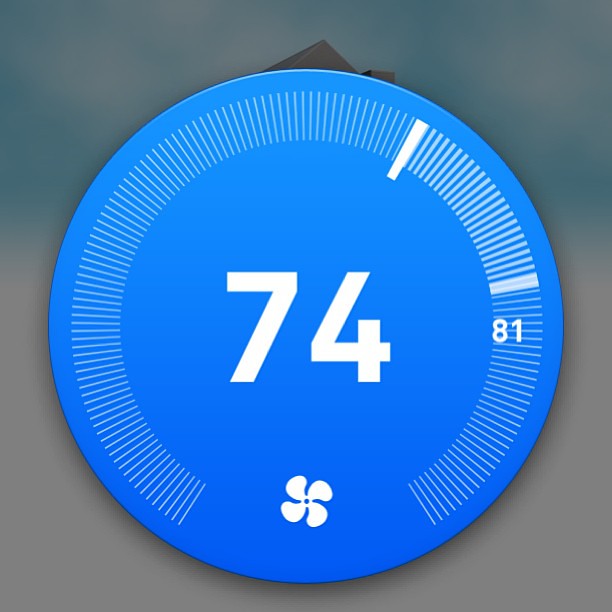The image depicts a minimalistic, squared-shaped digital interface, possibly from a smartphone app used to control a home thermostat. The background of the image features a gradient shading from light gray at the bottom to bluish-gray at the top, suggesting a cloudy sky behind a house. Visible at the top of this background is the peak of a roof and a small section of a chimney, giving the impression that the house is integral to the scene.

Dominating the central area of the image is a solid blue circle. At the center of this circle, the number "74" is prominently displayed in large, white digits, indicating a temperature setting. Beneath this number is a white icon resembling a fan or propeller, likely representing the cooling function of the thermostat.

Encircling the blue circle are small white dashed lines, with one needle-shaped, thick white line intersecting or overlapping them. On the right side of the circle, the number "81" is displayed in white text. This could indicate the current temperature, the target temperature, or another setting on the thermostat interface.

Overall, this detailed and neatly designed interface signifies a digital thermostat, most likely controlled via a smartphone application, allowing users to manage their home climate settings remotely.